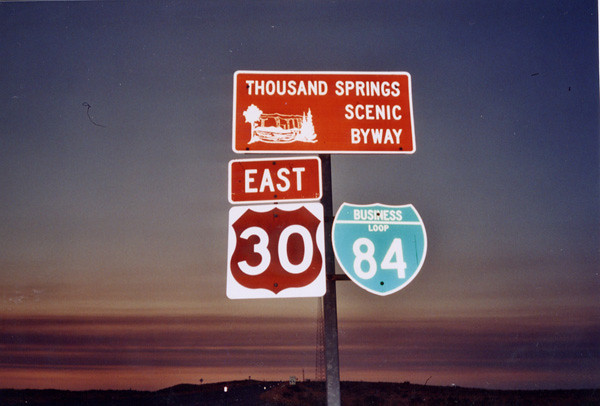This photo captures a series of street signs taken during twilight, either dawn or dusk. Each sign stands vividly illuminated against the semi-dark sky, suggesting the use of a flash. At the top, a rectangular sign proudly displays "Thousand Springs Scenic Byway" in white letters on an orange background, adorned with a small graphic depicting a scenic landscape. Just below, another orange sign with white letters prominently marks the direction "East". Further down hangs a shield-shaped sign indicating Route 30. Adjacent to these, a green and white shield sign denotes "Business Loop 84". All these signs are firmly affixed to a sturdy, gray metal pole positioned prominently in the foreground. The backdrop reveals a captivating horizon, where the dim light casts horizontal, multicolored stripes across the sky, transitioning into a deeper, dark blue expanse above.